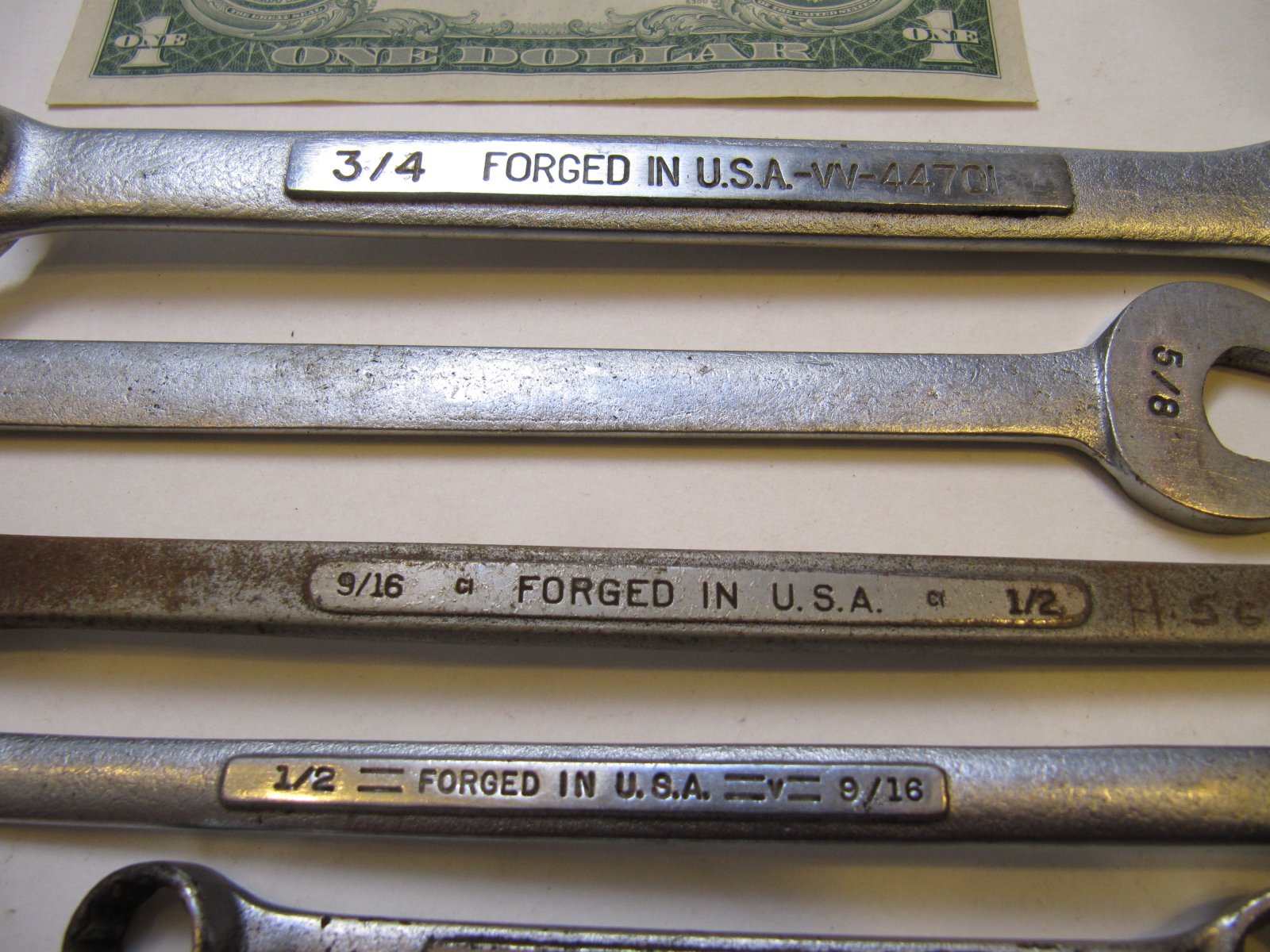This close-up photograph features a meticulously arranged row of five metal, open-end box wrenches, aligned horizontally from left to right against a buff-colored background. The image captures the central portions of the wrenches, revealing their sizes and a mixture of wear and rust textures. Each wrench is marked with its size and the inscription "forged in USA," with readable sizes including 3/4, 5/8, 9/16, 1/2, and 1 1/2. Notably, the wrench marked as 9/16 shows the most rust. Above the row of wrenches, at the very top of the image, is a partially visible upside-down U.S. one-dollar bill, displaying just the lower portion of the "ONE" text from its backside. The composition and lighting of the photograph highlight the texture and details of the metal surfaces, providing a rich visual contrast against the tan background.